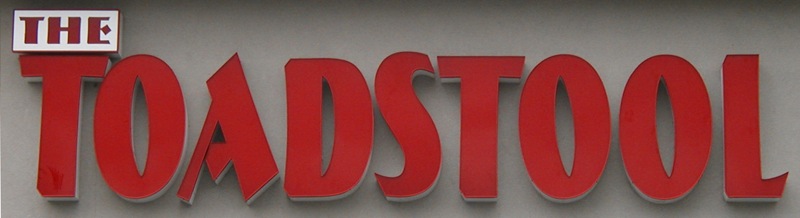In this image, we see a narrow, rectangular photo featuring a sign prominently displayed on a white wall. The sign reads "THE TOAD STOOL" in bold, red, block letters that appear slightly three-dimensional, with light gray edges adding depth to the text. A smaller sign, also in block letters, juts out from the wall above the "T" in "TOAD STOOL." This sign reads "B-T-H-E" and maintains the same red lettering against a white background. The wall, though appearing white, has dark gray shadows and linings that suggest the image is not brightly lit, contributing to a somewhat atmospheric and subdued appearance.